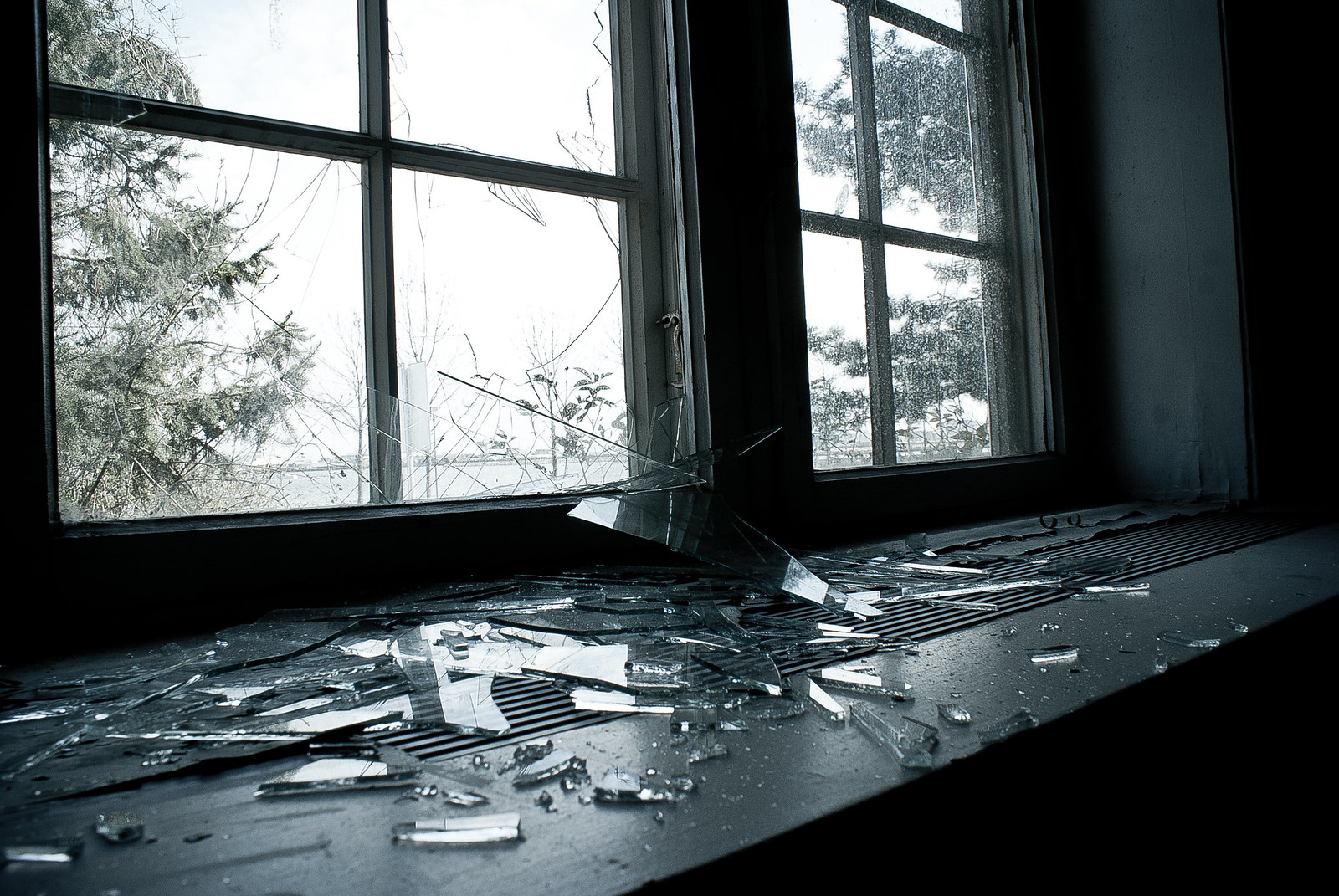The image depicts a broken window situated on the left side of a set of windows divided by brown-blackish bars. Each window section appears to be divided into at least five smaller panes. The broken window, primarily affecting the top right and bottom left sections, also shows cracks extending into the other two sections, with the glass shattered inward onto the window sill. The sill and the surrounding wood frame are painted black and covered with shards of glass varying in size from small to large, all appearing sharp and jagged. Behind the broken window, the room is very dark, and through the intact, wet panes, a gray, rain-soaked sky and trees in the background are visible. The windowsill also features a decorative vent-like structure, possibly made of a smooth wood material.